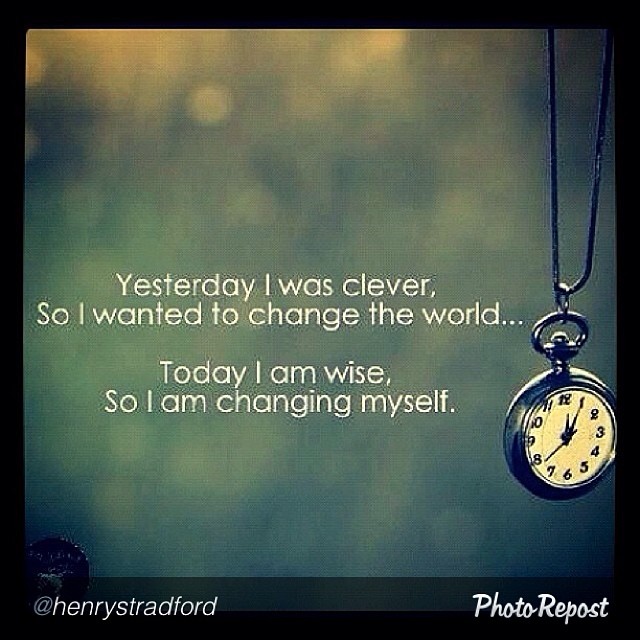This image is an inspirational poster set within a square black border. The background features a heavily blurred mix of green, blue, gray, and yellow hues, creating a soft, diffused light effect. On the right side of the image, a silver pocket watch dangles from a black cord, showing the time as 12:05. In the center, the poster displays a motivational quote in white text: "Yesterday, I was clever, so I wanted to change the world... Today, I am wise, so I am changing myself." The attribution "At Henry Stratford, S-T-R-A-D-F-O-R-D" is displayed in the bottom left corner, while the words "Photo Repost" appear in a cursive white font in the bottom right corner.